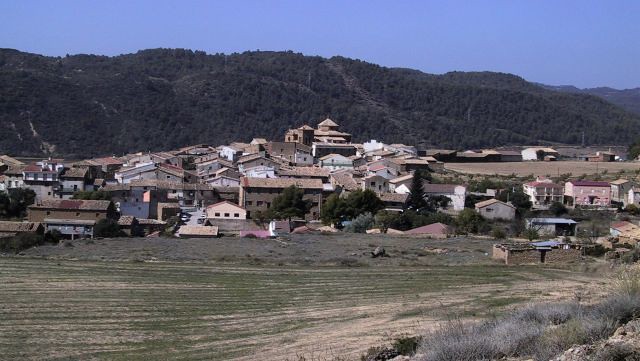The photograph captures a picturesque scene from an elevated vantage point on a hill, looking down at a cluster of houses with their varied rooftops. Set against a backdrop of lush, tree-covered hills, the surrounding landscape is predominantly green, indicating a warm time of year. The sky above is a gradient of blue, ranging from light to dark, and is cloudless, contributing to the serene atmosphere. 

In the foreground, there appears to be a small park or open area with patches of grass that vary in color from green to brown and tan, hinting at a mix of maintained and more natural, untamed growth. A solitary barbecue stands out amidst this grassy expanse, devoid of any people or other identifying elements. The overall scene is residential, with an absence of commercial buildings, underscoring a sense of tranquil suburban or rural life. The photograph gives a sense of distance from both the homes and the surrounding natural beauty, capturing the expansive and quiet charm of the area.